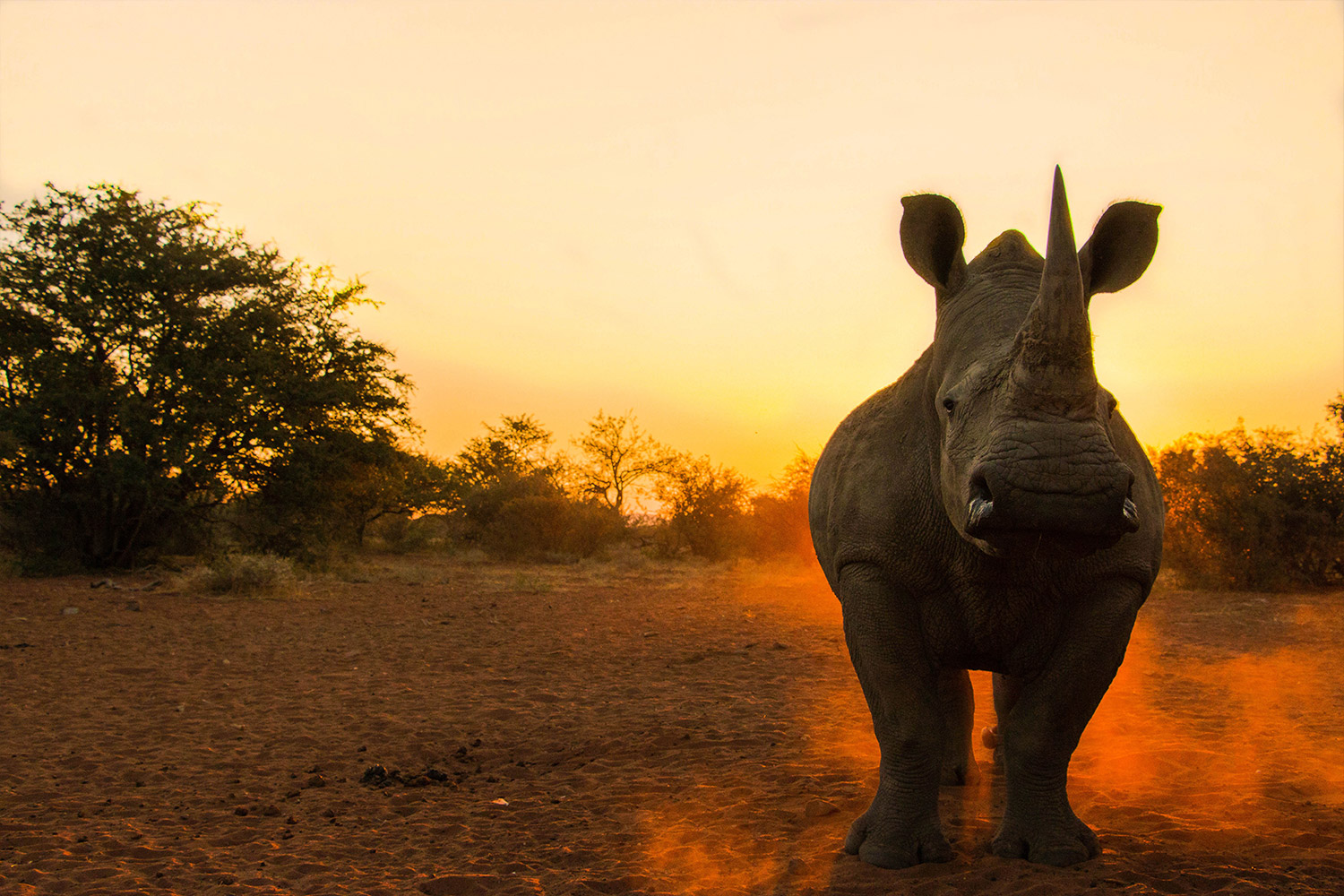This breathtaking photograph captures a rhinoceros standing majestically on the African savannah at sunset. The rhino dominates the right side of the composition, facing the camera, with its horn prominently visible and its eyes staring directly ahead. The animal's body casts a shadow that creates a glowing, vibrant red and orange dust cloud around its feet, illuminated dramatically by the sun positioned directly behind it. 

The left side of the image is noticeably emptier, featuring a barren landscape of sand interspersed with sparse shrubs and set against a background of savannah trees and bushes. The sky above is a dull gray, devoid of stars and sun, adding a stark contrast to the vivid scene below. The overall color palette of the image is suffused with warm tones of orange and peach, lending it a surreal quality. Despite the darkness creeping in, the greenery of some bushes is still visible, and the trees appear as dark silhouettes against the setting sun, enhancing the focus on the rhino as the central figure of this striking and beautifully composed scene.